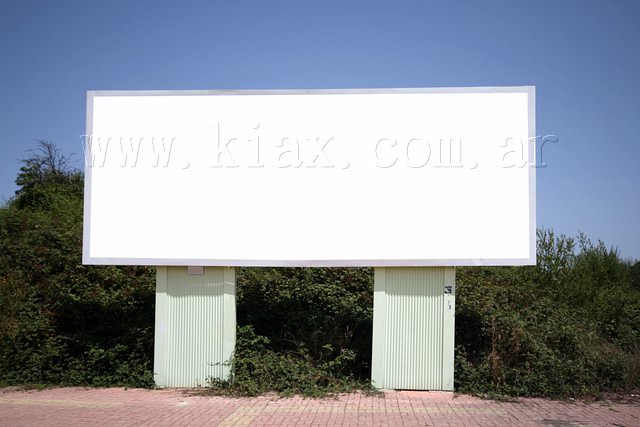A large white board, resembling an oversized classroom piece, stands prominently against a backdrop of lush, beach-like vegetation. The board is anchored by two pale green supports that resemble unconventional doors. In front of it, a brick sidewalk showcases a variety of light-colored bricks, adding texture and visual interest to the scene. Above the board, a watermark with the URL "www.keaxe.com.ar" is visible, but not part of the actual physical setting. The clear blue sky provides a pristine and vibrant overhead expanse, framing this intriguing composition.